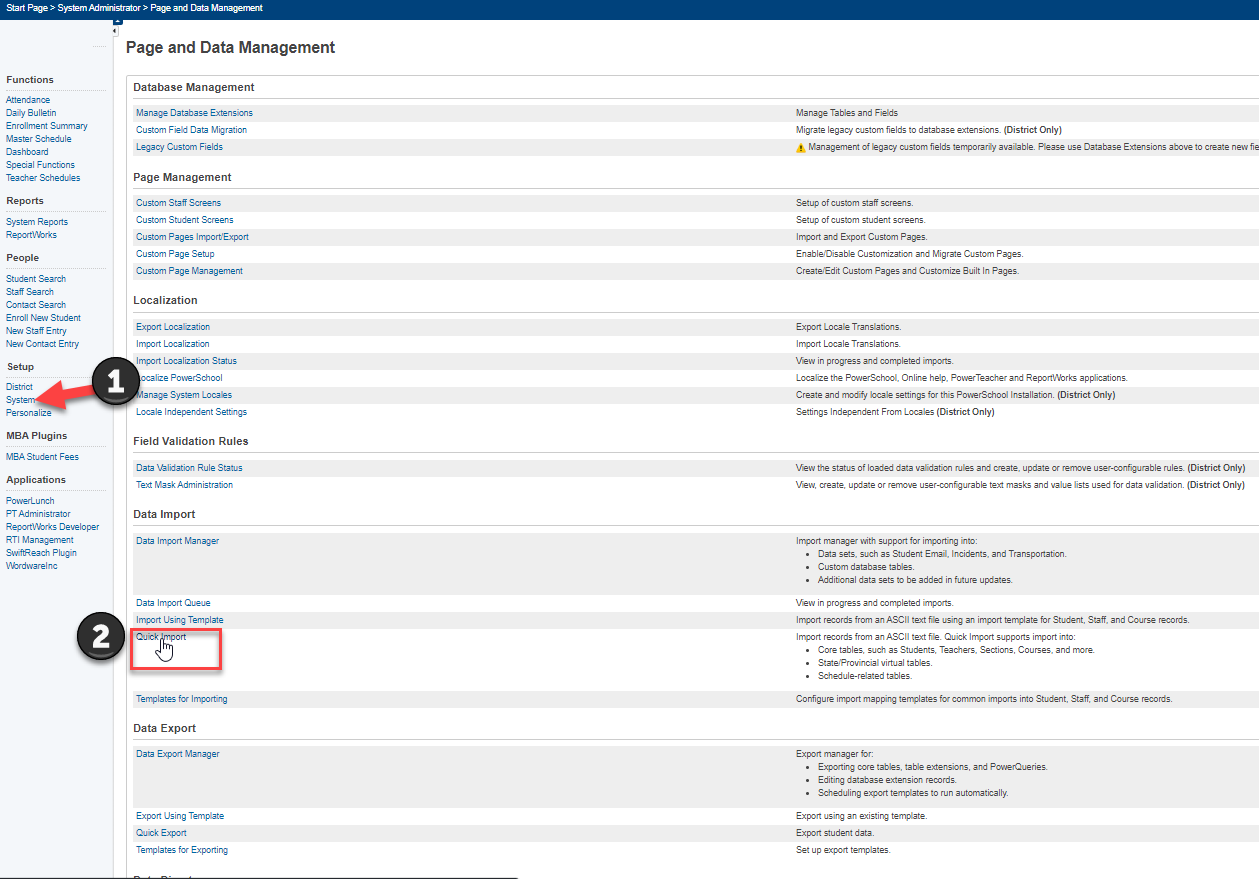The image appears to be a detailed view of a start page tailored for a system administrator within a WordPress-like content management interface. It prominently features a header highlighted by a thin blue line with the words "Page and Data Management" clearly displayed and selected. The setup consists of a comprehensive menu on the left side, divided into sections with the primary headers in black reading: Functions, Reports, People, Setup, MBA Plugins, and Applications. 

Under the "Setup" section, a red arrow points to the second sub-option, which might relate to system settings, accented by a large number "1" inside a gray circle with a black outline adjacent to it. The screen's main workspace is devoted to "Page and Data Management", offering a variety of sub-options. The top options are grouped with alternating pink or gray and white lines, aiding readability. The list includes "Manage Database Extensions," "Manage Tables and Fields," "Database Management," "Page Management," "Localization," "Field Validation Rules", and "Data Import." Notably, "Data Import" has a sub-option numbered "2" (likely "Quick Import") that is selected, notable due to a hand cursor hovering over it. This intricate layout is packed with textual information, appearing balanced meticulously for effective navigation.